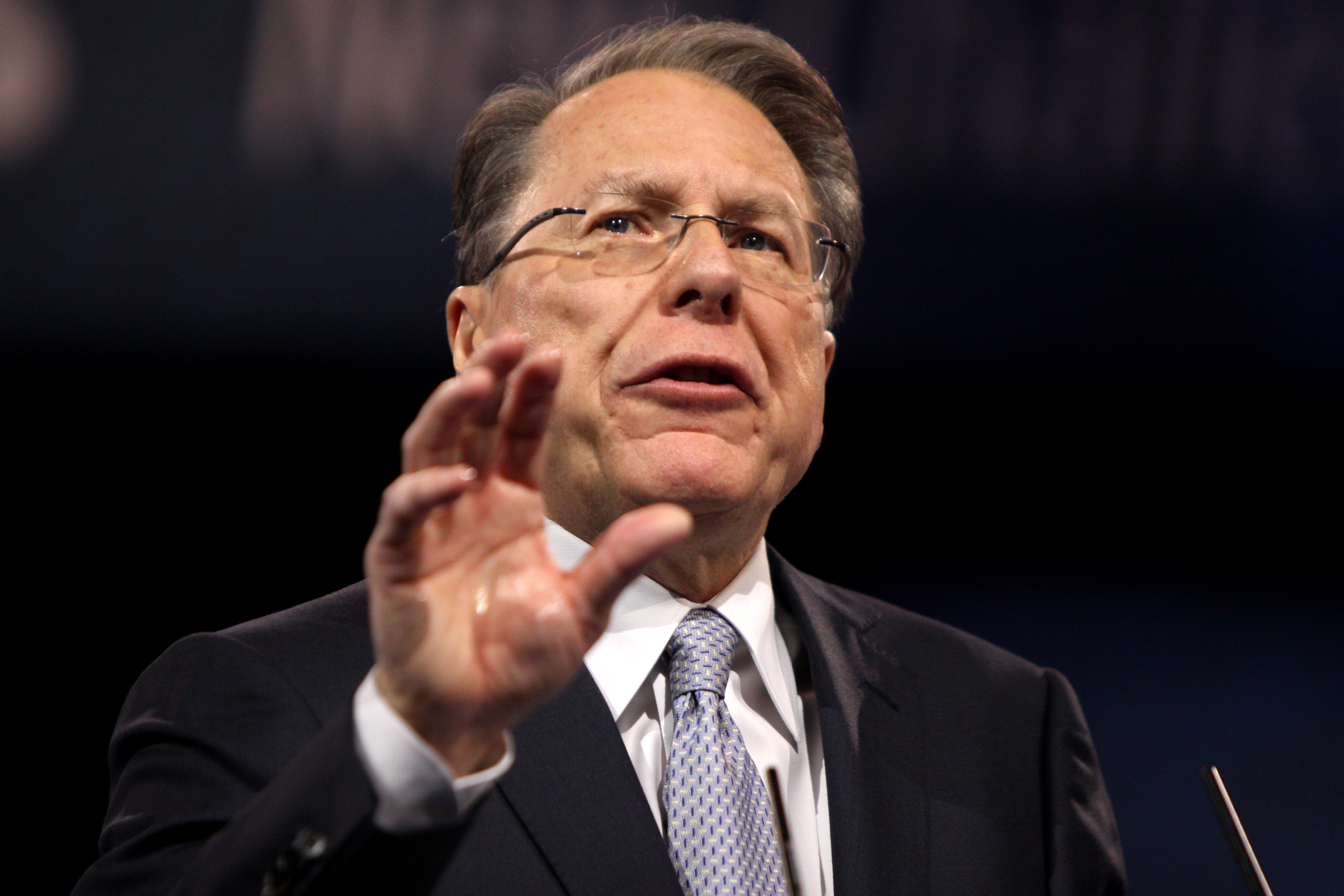The image features an older man with short, brownish-gray hair combed to the right without any visible gel. He is wearing frameless thin glasses and has dark blue eyes. His face is serious and his mouth is slightly open, as though he is speaking. Dressed in a dark gray or black suit jacket with a white collared shirt and a light blue tie adorned with white patterns, he stands with his right hand extended upward, palm open, seemingly addressing an audience. A small microphone is visible to the left side of the picture, implying he is at a podium. The backdrop is a dark blue or black color, and there are blurred streaks of light or possibly a curtain in the upper left-hand corner.